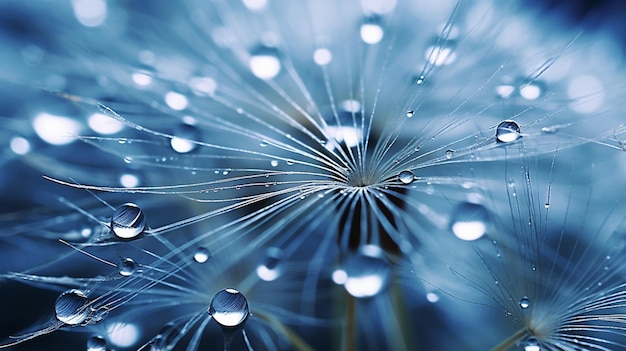This is a striking, full-color close-up photograph, professionally captured under either artificial or natural light, showcasing an exquisitely detailed dandelion fluff adorned with water droplets. The horizontally rectangular image highlights a complex interplay of colors, primarily blue, white, black, and shades of gray, with water droplets serving as tiny magnifiers. The fluff's thin, white filaments radiate from the center, extending in all directions and carrying these perfectly round droplets, which exhibit a slight blue hue. The lower left and upper right corners contain some black patches, while the bottom and edges of the image are slightly blurred, emphasizing the sharp, focused center where the intricate details of the dandelion and water droplets are most prominent.